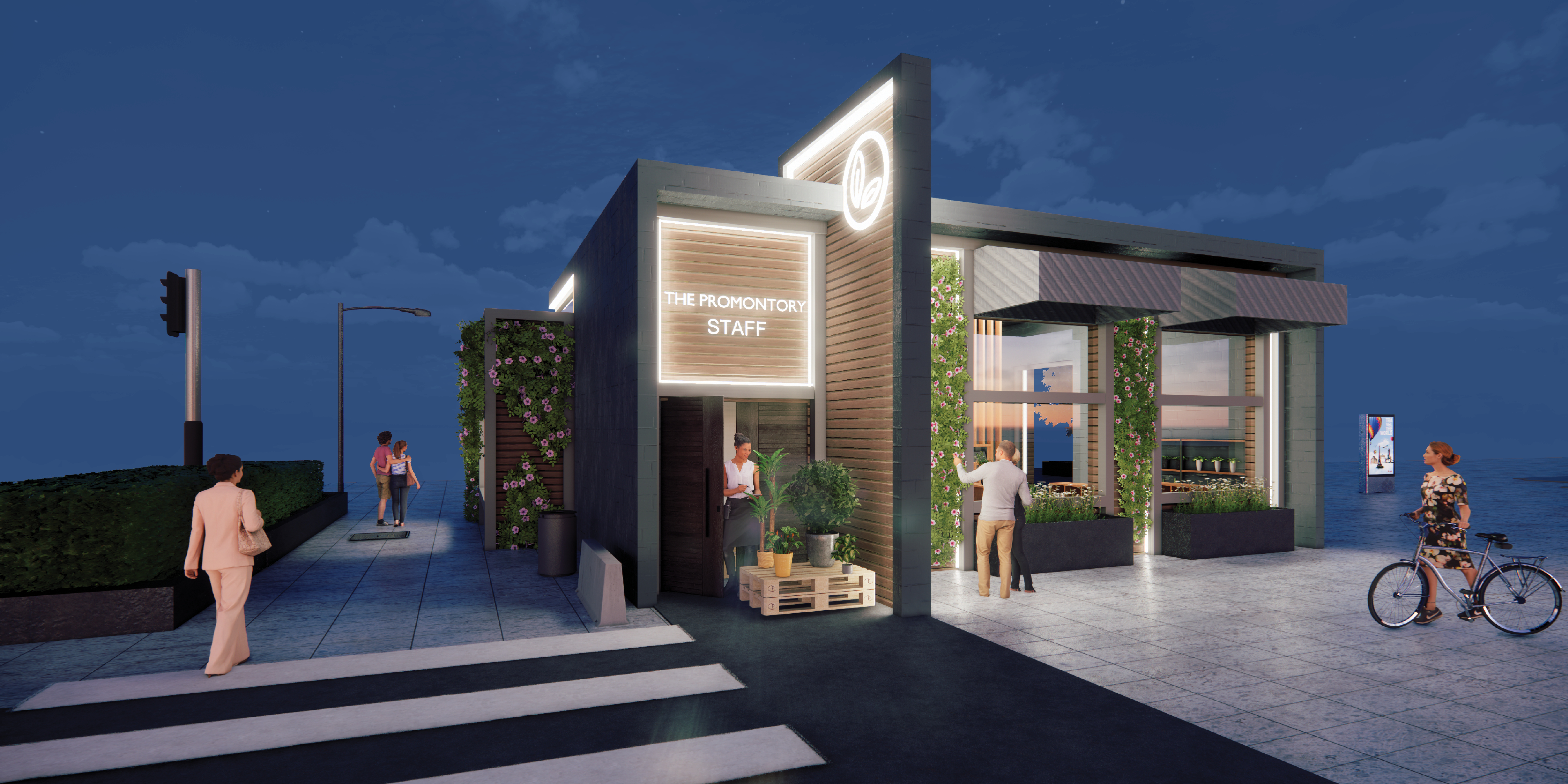The animated image, likely AI-generated with a cartoonish aesthetic, depicts a night scene characterized by a very dark blue background with some dark blue clouds. On the left side, there's a distinctive walkway with black and white horizontal stripes adjacent to a more traditional gray-tiled pathway. A streetlight illuminates two people walking arm-in-arm beneath it. A stoplight can be seen to the left of a woman in a light pink suit holding a purse. Both real-looking people and the environment seem artificially created, suggesting computer-generated imagery.

To the right, there's a modular-style building labeled "The Promenatory Staff" in bright white on a light brown sign. The building, with large windows and overhangs, is embellished with concrete planters and wood siding designed for growing plants. Below the sign, there are plants and a woman nearby. Another area showcases a light gray tiled walkway where a woman in Nike shoes and a dress gazes at a store while holding a bicycle.

Around the scene, more individuals populate the area, including a lady in an apron tending to plants on a pallet and a couple embracing and admiring flowers. The scene blends realistic human figures with a stylized, computer-generated environment, underscoring its likely origins in digital design software or video game graphics.